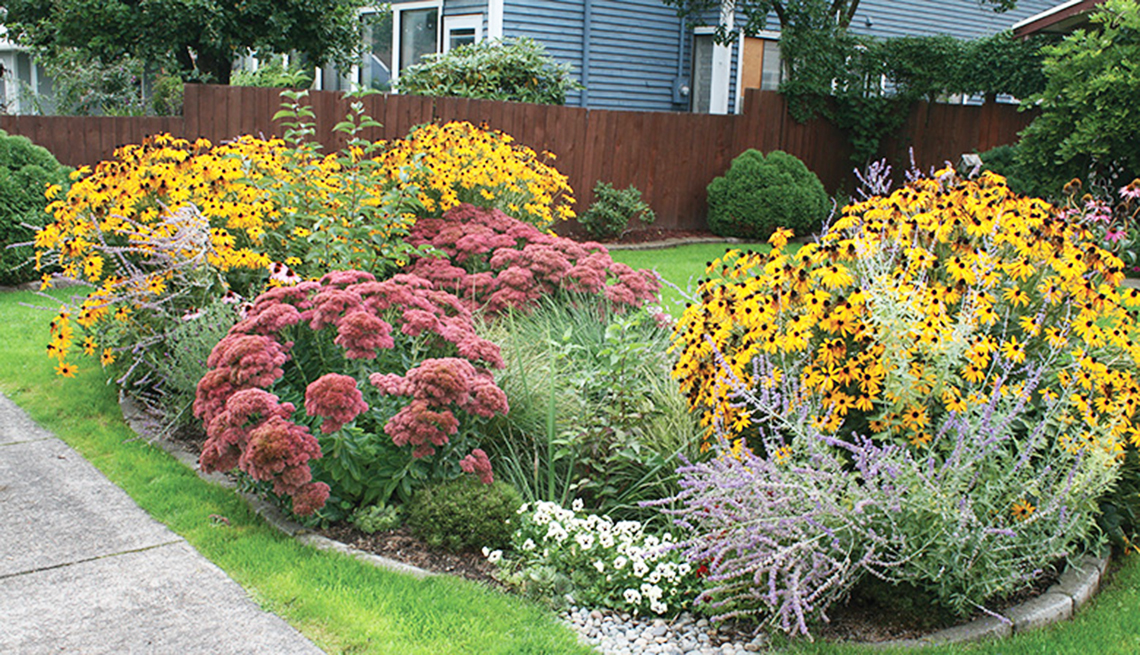This photograph captures a lush garden in someone's backyard, brimming with vibrant colors and intricate details that evoke a summertime setting. The focal point of the scene is a large, oval-shaped brick garden bed, bordered with elongated gray stones. The garden is teeming with an array of flowers, including tall purple blooms with full heads, yellow daisies with dark centers, smaller white flowers, and vibrant red flowers, all interspersed with greenery. Surrounding the garden bed is a verdant, well-maintained grassy yard.

In the left foreground, a cement sidewalk slopes from the bottom left corner upwards, guiding the viewer's eye towards the background. Dominating the background scene is a wooden stockade fence, dark brown in color, which seems to define the property's boundary. In front of this fence, neatly trimmed green shrubs are arranged in rounded shapes. The backdrop includes a blue-sided house with white trim around the doors, partially obscured by the greenery. Additional visual interest is provided by a tree on the right side of the image and another on the far left, adding to the garden's rich, natural ambiance.